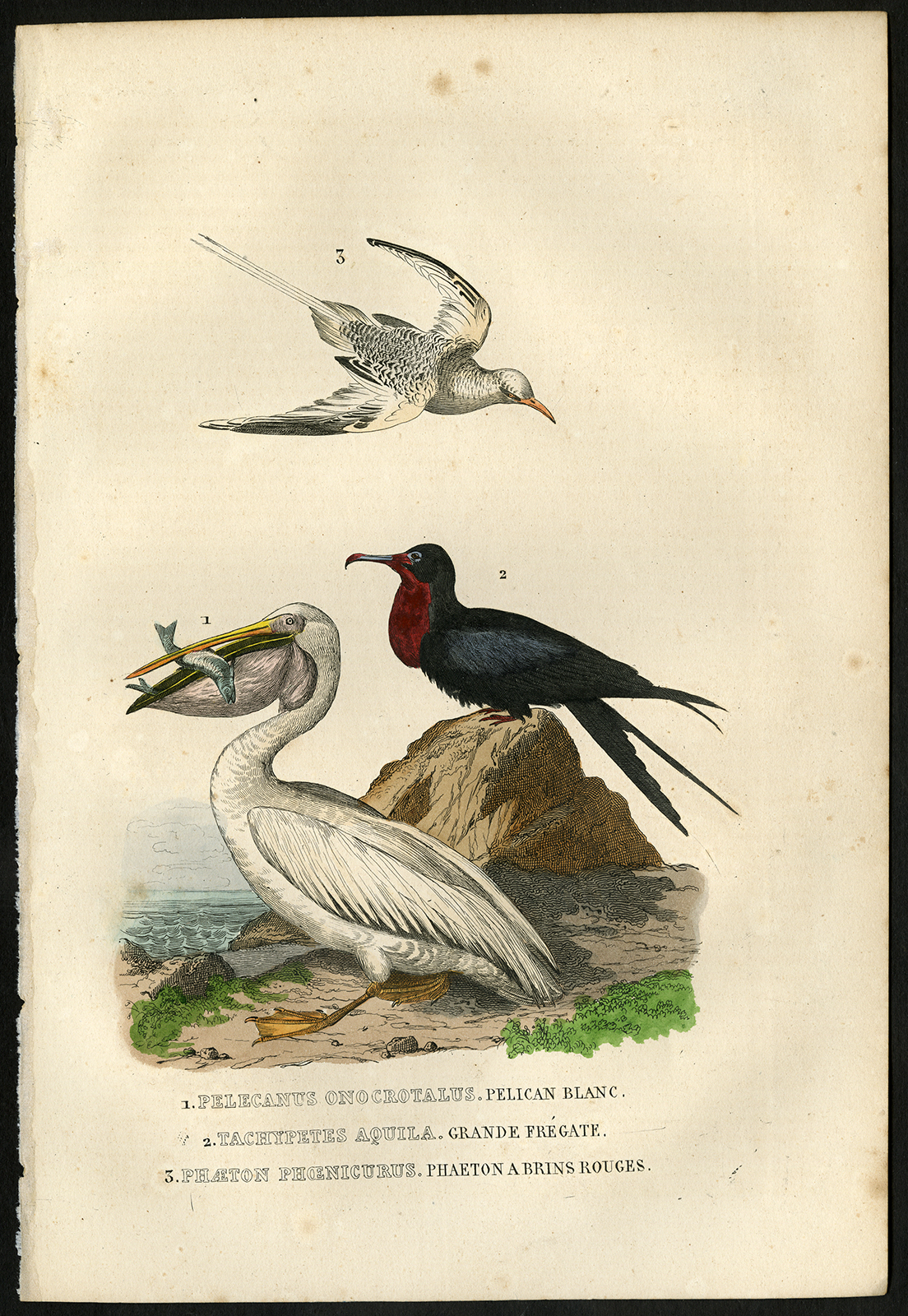The image appears to be an antique illustration from a vintage book, displaying three uniquely detailed birds against a beige, slightly stained background that shows its age. At the top of the illustration, there's a bird in mid-flight, identified as *Phaeton phaenocurus*, commonly known as the red-billed tropicbird, characterized by its white and black feathers, orange beak, and long, pointy tail. This bird is labeled with the number 3.

Below it, perched on a rock, is a *Tachypetes aquila*, or great frigatebird, labeled with the number 2. This bird is notable for its black plumage and distinct red throat.

On the ground, there is a white pelican, identified as *Pelecanus onocrotalus* (great white pelican), holding a fish in its beak and labeled with the number 1. Below the illustration, the birds are further described with their scientific names and additional text, possibly in another language, providing educational information about each species. This detailed composition captures the essence of ornithological studies from a bygone era.